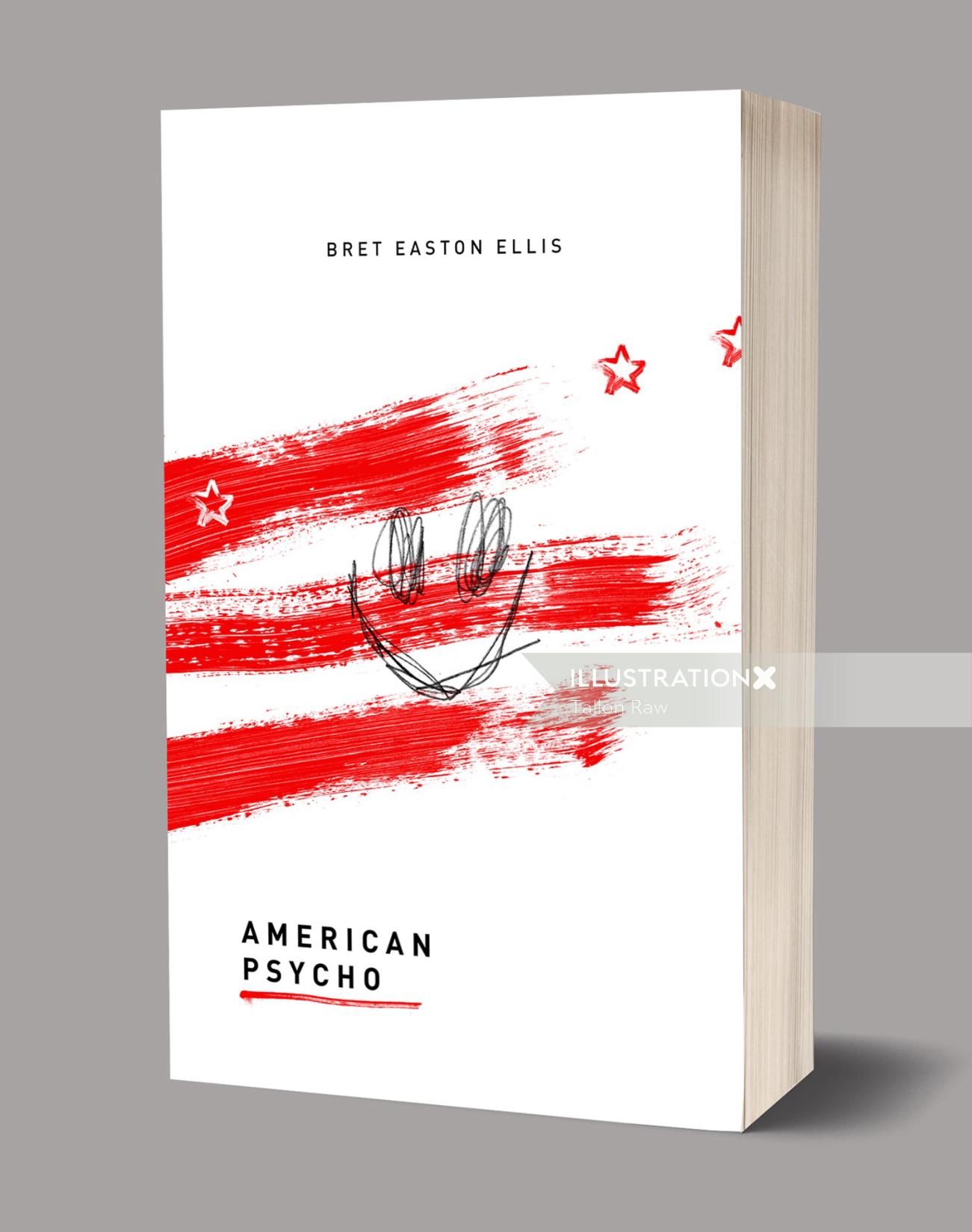The photograph showcases a book positioned upright and slightly tilted, centered against a light gray background with a darker gray drop shadow on its right. The book cover is predominantly white with striking red elements and black text. The top of the cover features the author's name, "Bret Easton Ellis," in bold black letters. Dominating the cover are three red stripes resembling smeared blood, incorporating three red stars on the top stripe and a crudely drawn black smiley face with squiggly eyes and a curved mouth in the center. Below, the title "American Psycho" is displayed in black font, underlined in red. The book's right side shows beige-colored pages. In the middle right of the image, a translucent gray banner with the white inscription "Illustration X" adds a subtle detail. Overall, the design implies a raw, intense aesthetic, echoing the themes and graphic elements associated with the novel.